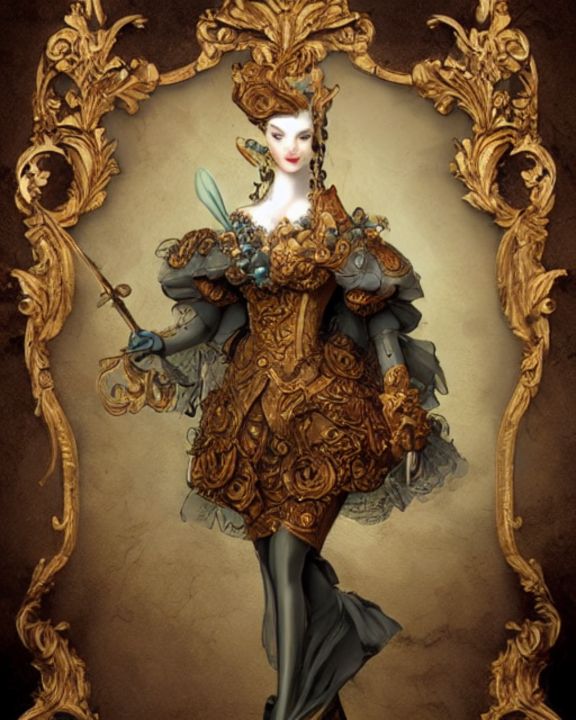In this artist's detailed depiction, a woman is portrayed standing centrally within a vertical gold leaf frame. Her face, marked by pale white skin, gives off an almost ethereal aura, with a slight, intriguing disfigurement. The backdrop transitions smoothly from light to dark brown, emphasizing her presence. She's attired in an elaborate, old-fashioned golden dress with intricate beading and floral embellishments, reminiscent of a bygone royal era. The dress also features gray arm material, dark gray leggings, and hints of green. Her flowing red hair is styled with a grand headdress that seamlessly connects to the frame's upper edge, adding a touch of regality. Additionally, she holds a gold sword, enhancing the picture’s opulent and historical feel.